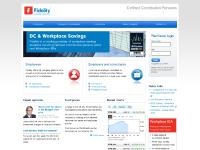The image appears to be a slightly pixelated and blurry information card or document with a predominantly gray and white color scheme. It features a white square at the center top with the word "Fidelity" situated in the upper left corner. To the left of this square is an orange rectangle containing the letter "F". Below this, various sections containing blue titles followed by black text are difficult to read due to the blurriness. 

On the bottom left side of the image, there is a small photograph of a man with light-colored, possibly gray or blonde hair, and glasses, suggesting he might be the subject or author of the document. On the bottom right side, there is a small red rectangle with text inside it, next to a poorly visible graph or chart. The background of the image transitions from gray at the top to white at the bottom, creating a gradient effect. Overall, the details are obscure, making the content hard to decipher.